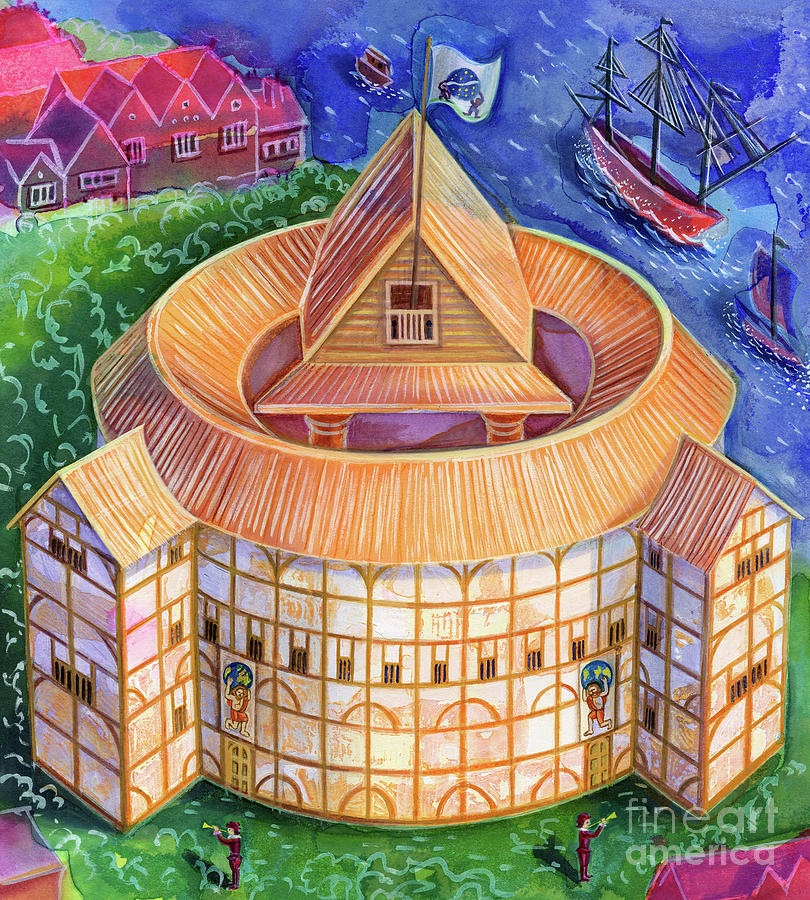The painting depicts a vivid daytime scene outdoors by a harbor. Dominating the foreground is a large, circular theater, reminiscent of the one Shakespeare used to perform in. This round building features two rectangular side buildings with gabled, slanted roofs. The central structure boasts an A-frame gabled roof atop a wooden platform. Above, flags wave, one of which appears to display a blue crab or similar creature.

Fronting the theater, on a stylized green lawn, stand two men in red outfits and hats, each blowing into a trumpet. These trumpeteers are stationed near the doors of the theater, facing outward.

The building's façade is adorned with a gridwork of painted panels, including depictions of Atlas bearing the globe above the doors. Surrounding the main theater is a collar of orange and white vertical lines extending from the roof downwards. To the right of the building lies a body of blue water, where two sailing ships navigate from the bottom right to the top left. Additional elements include numerous red-roofed houses in the background and a scattering of smaller structures at the bottom corners of the painting. Text at the bottom right of the image reads "Fine Art America."